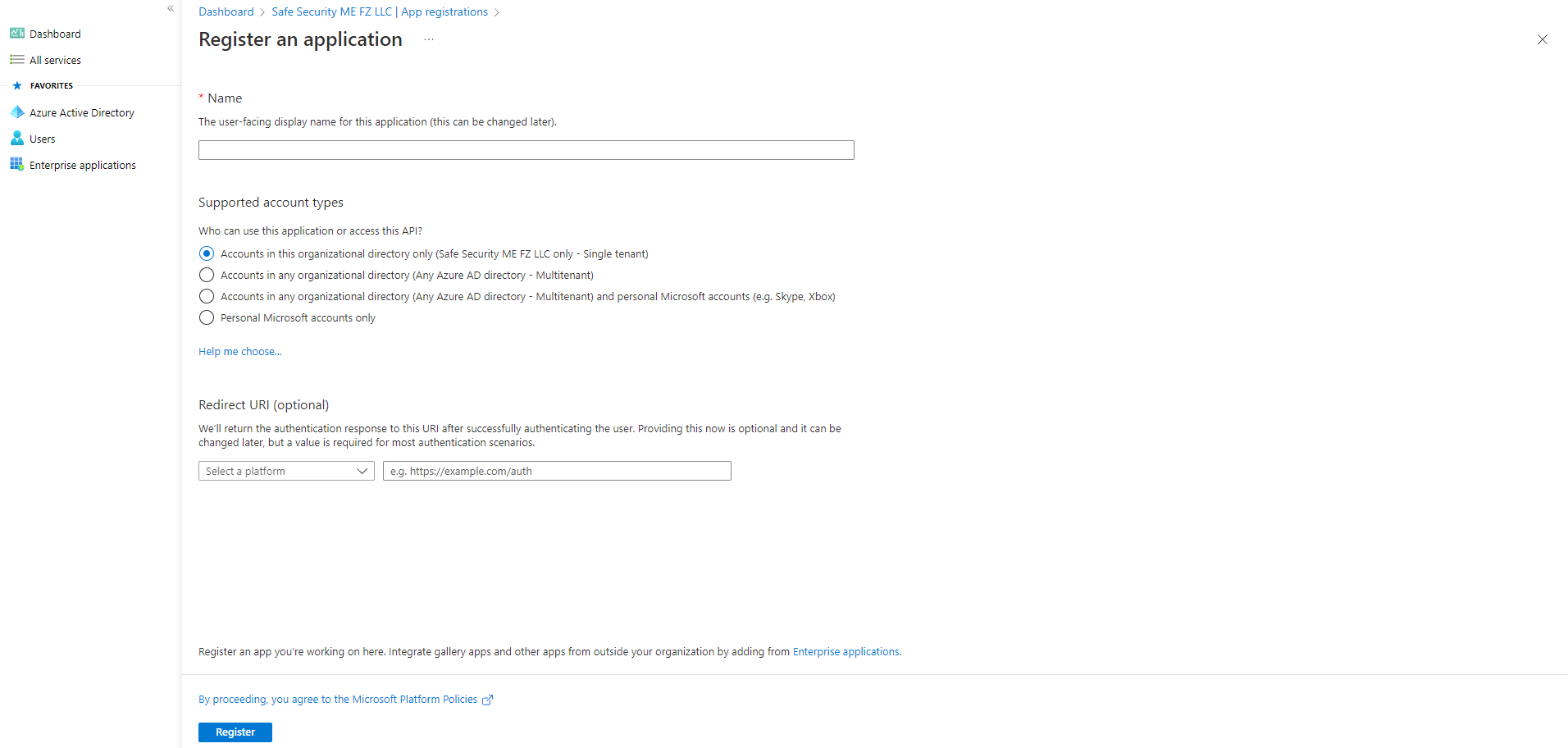This image is a screenshot from an undisclosed website, likely a user interface within Microsoft Azure's portal, featuring several navigational and functional elements related to application registration. 

On the left side of the screenshot are clickable sections organized into a vertical sidebar, listing options such as:
- Dashboard
- All Services
- Azure Active Directory
- Users
- Enterprise Applications

On the main section to the right, the heading "Dashboard" appears, accompanied by a navigational arrow pointing to "Safe Security under MEFZ LLC." Below this, there is an "App Registrations" section.

The detailed "Register an Application" form is presented prominently. It includes the following components:
- **Name:** Input field for the user-facing display name of the application, currently blank, with a note that the name can be changed later.
- **Supported Account Types:** Options to specify who can use or access the application:
  - "Accounts in this organizational directory only (Safe Security MEFZ LLC only - Single tenant)" - This option is currently selected.
  - "Accounts in any organizational directory (Any Azure AD directory - Multi-tenant)"
  - "Accounts in any organizational directory (Multi-tenant) and personal Microsoft accounts (e.g., Skype, Xbox)"
  - "Personal Microsoft accounts only."
  A "Help me choose" link, indicated in blue, provides additional assistance for selecting the appropriate account type.

- **Redirect URI (Optional):** Explanation that the URI will receive the authentication response upon successful user authentication. Although optional at this stage, it is required for most authentication scenarios. A dropdown to select the platform includes a placeholder example "https://example.com/AUTH."

Additional guidance states:
- **Register an App:** Prompts to register the application currently being worked on.
- **Integrate Gallery Apps:** Advises on adding enterprise applications from within or outside the organization, with "Enterprise Applications" being a clickable blue hyperlink.

Finally, there is a call-to-action with a blue "Register" button featuring white text. A note underneath this reminds users that by proceeding, they agree to the Microsoft platform policies.